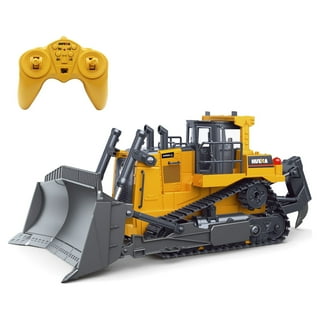The image features a brightly colored yellow toy bulldozer with a detailed design, including a large, curved gray plastic shovel at the front and black hitch and tires. The bulldozer has tracks that wrap around multiple wheels, with visible silver vents emerging from the top where the engine is located, and a black apparatus attached to the rear along with a small red button. In the upper left corner, a yellow remote control resembling a gaming or PlayStation controller can be seen. The remote has two prominent buttons for up and down movements, four additional yellow buttons, and several smaller black buttons. Both the bulldozer and the controller are set against a plain white background, highlighting their vivid colors and fine detail, making it evident that this toy, reminiscent of every child's dream, is designed for interactive play in a toy room setting.